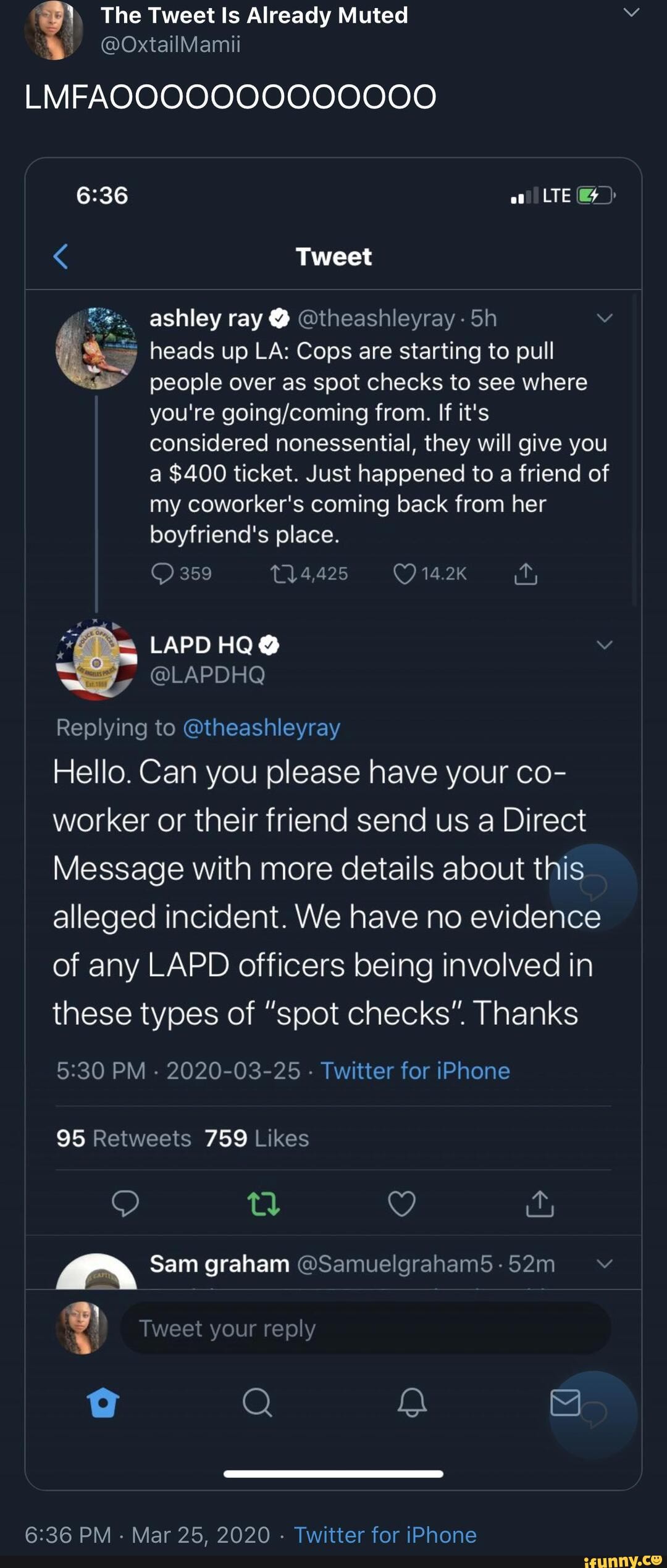A screenshot from a phone displaying a Twitter post occupies the frame. The status bar at the top is absent, missing the usual time, network, and battery indicators. On the top left, there's a profile icon featuring a girl with long brown hair, wearing a black dress. The text next to it reads, "LMFAO," followed by "636" in white letters and "LTE" with two bars indicating signal strength, and a battery at less than 50%.

The tweet, posted by Ashley Ray, reads:
"Heads up LA, cops are starting to pull people over for spot checks to see where you're going/coming from. If it is considered non-essential, they will give you a $400 ticket. Just happened to my friend's coworker coming back from her boyfriend's place."

Below this, the LAPD has replied:
"Hello, can you please have your coworker or their friend send us a direct message with more details about this alleged incident? We have no evidence of any LAPD officers being involved in these types of spot checks. Thanks."

This tweet has garnered 95 retweets and 955 likes. An obscured reply from another user named Sam Graham is partially visible beneath the interaction metrics. Further down is an input field labeled "Tweet your reply" next to the original poster's profile image.

At the bottom, the navigation bar typical of Twitter interface is seen, and a timestamp indicating "6:36 PM - March 25, 2020 · Twitter for iPhone" is displayed. The background throughout the image is black.